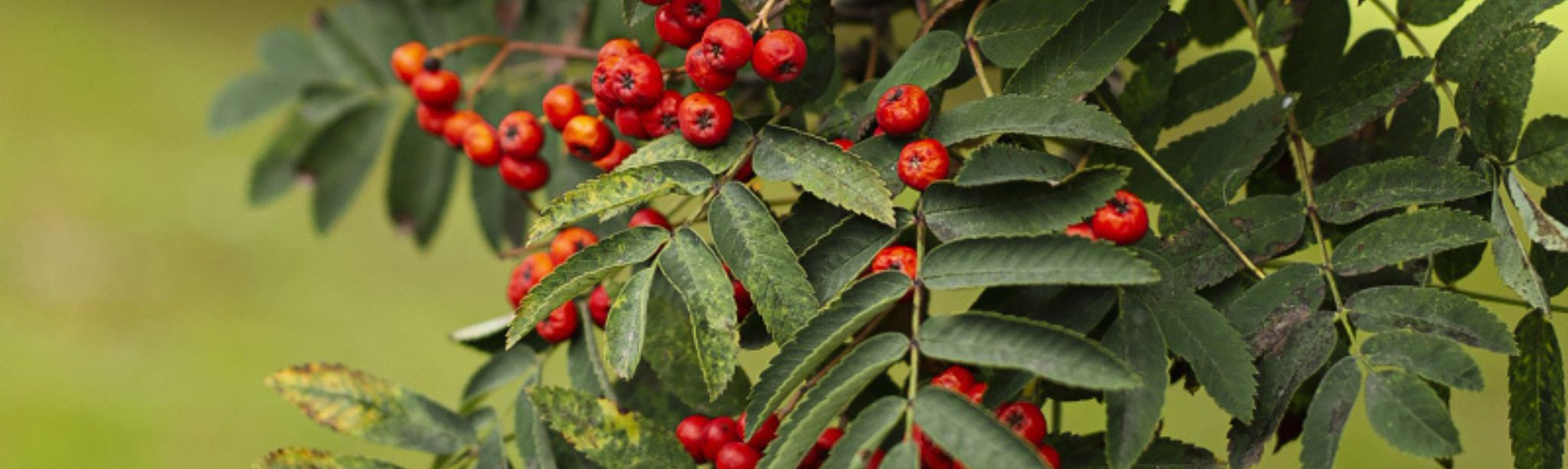The image showcases a cluster of vibrant, round red berries, reminiscent of cherry tomatoes, with a characteristic six-segment star at the bottom of each berry. The berries, positioned near the center of the image, are attached to a plant with long, narrow green leaves that feature serrated, zigzag edges. Some leaves exhibit a yellow or brown hue, indicating signs of aging or damage, while others remain lush and green. The plant's tiny branches are scattered with these elliptical leaves. The photograph, taken in a wide, landscape orientation, has a background of blurred green and brown hues, emphasizing the bright red berries and the intricate leaf patterns in the foreground. The overall style of the image is photographic realism.